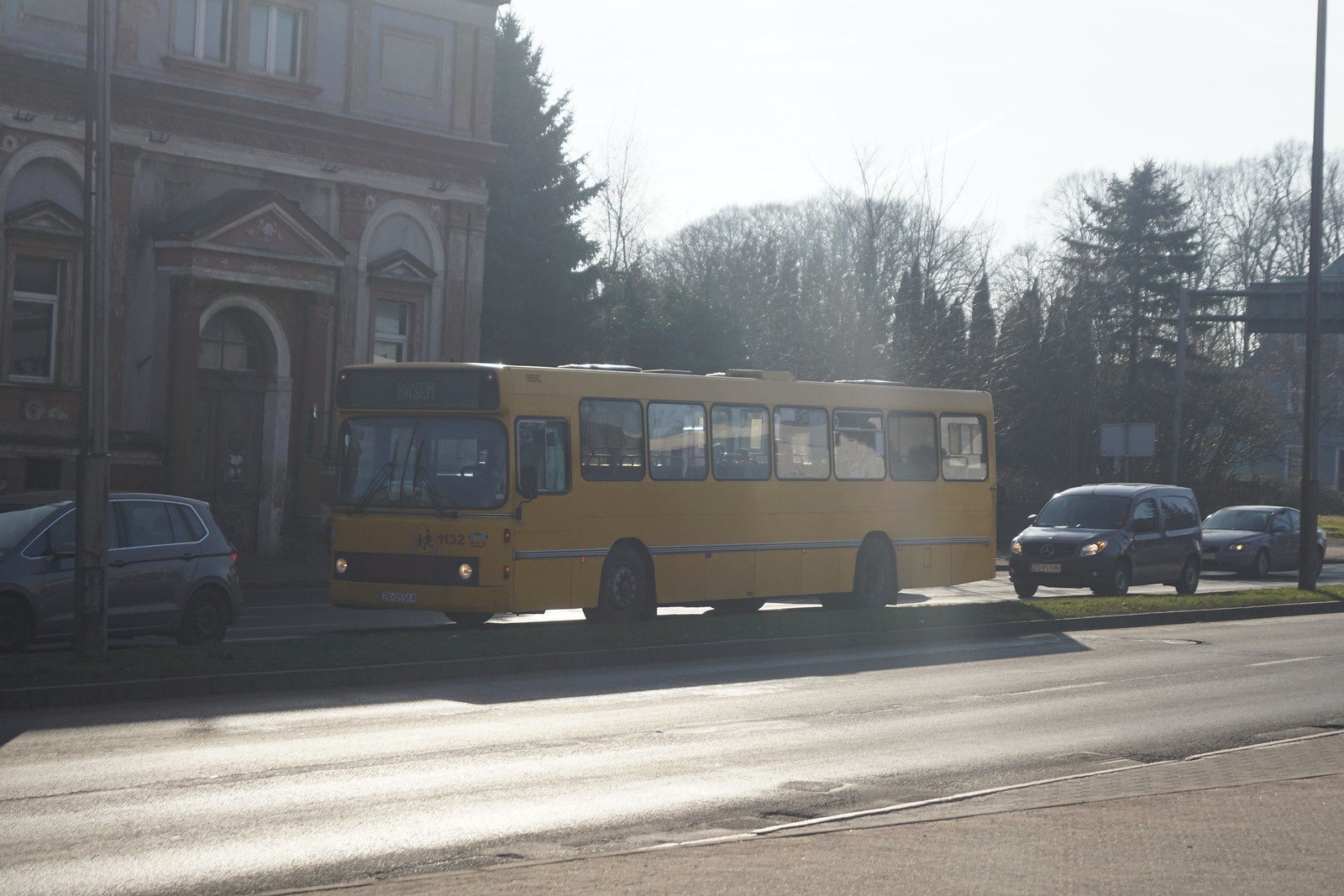This photograph depicts an older, yellow school bus with the identifier "1132" and an illustrated sign of schoolchildren walking. The bus is parked on a sunlit two-lane roadway in front of an older, neoclassical building that could be a church or a school, characterized by a peaked roof, arched inset green door, and tall peaked windows. The façade of this historical building is complemented by a small line of modern cars: a gray car in front of the bus, and a black minivan with its lights on behind it, suggesting they might be queued together, potentially exiting a parking lot. The sun shines brightly from above and behind the bus, casting light on the roadway and partially on the cars. Trees and a hint of a blue building in the distant background add to the scene, which, despite the bright sun, gives off a wintry feel.